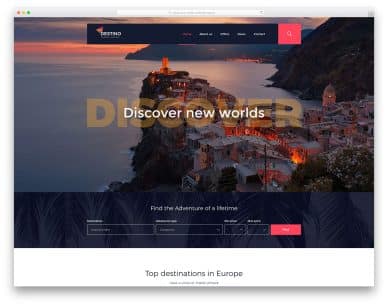In this image, a webpage is displayed with a prominent search button. The backdrop features a panoramic view of a cityscape overlooking the sea, framed by distant mountains. At the center of the image, bold text reads "Discover New Worlds." Additional informative text includes phrases such as "Top Destinations in Europe" and "Find the Adventure of a Lifetime." The design palette includes vibrant shades of orange, red, blue, yellow, and gray, adding to the vivid and inviting visual appeal.